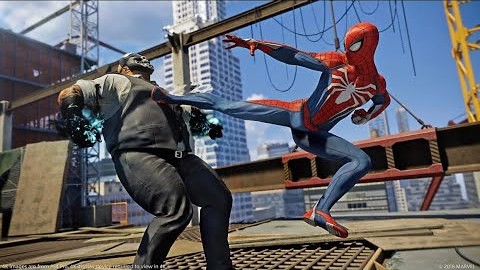In this dynamic scene set against a bustling construction site, Spider-Man takes center stage. He is clad in his iconic costume—blue pants paired with red and blue shoes, and a red and blue top featuring a prominent white spider emblem on his chest. His mask, detailed with large black-rimmed eyes, heightens his fierce look. With one arm outstretched for balance, Spider-Man delivers a powerful kick to a hulking adversary. The massive foe, dressed in dark overalls secured by a hefty belt, stumbles backward from the force of the attack. He wears a gray shirt beneath his overalls, adding to his rugged appearance. The backdrop features a sprawling construction site, with a substantial concrete structure and beams crisscrossing the scene. Towering skyscrapers and a clear blue sky frame this intense moment, capturing the essence of urban action and adventure.